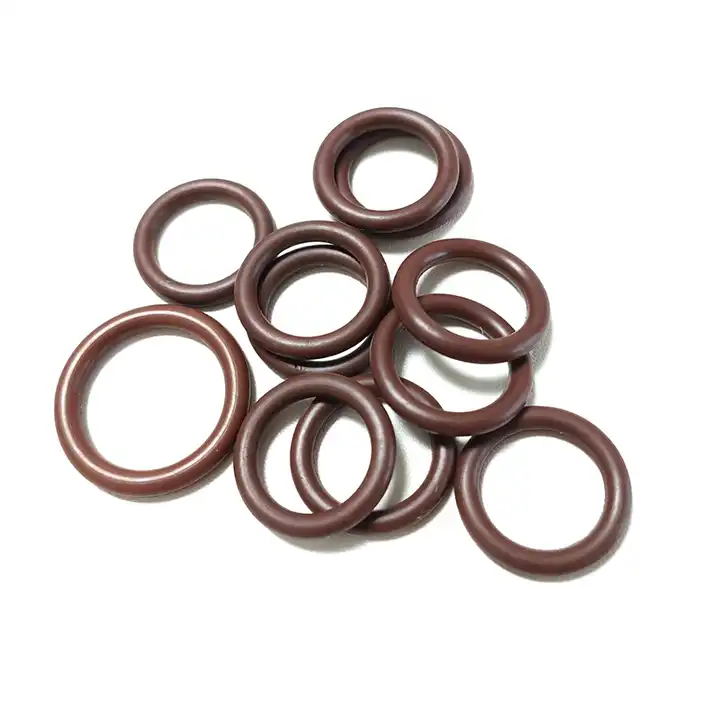The photograph depicts a collection of brown plastic rings on a white background. Most of the rings are a shiny, reddish-brown color, resembling old-fashioned drapery hanging rings, but they seem to be made of plastic rather than wood due to their perfect appearance. There are eleven rings in total: ten smaller rings and one larger ring, lighter in color, situated on the left-hand side. The rings are arranged in a somewhat haphazard manner, with some piled directly on top of others, creating a loose, triangular formation. The rings cast subtle grayish shadows on the white surface beneath them, enhancing the depth and texture of the image. The camera angle appears slightly elevated, as if the shot was taken from directly above the rings.